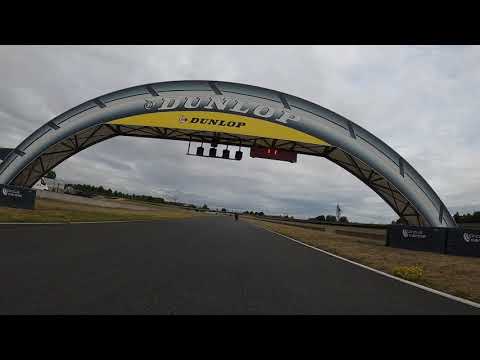The image depicts a European-style Formula One racetrack with a broad, asphalt track flanked by grass on both sides. Prominently featured is the iconic Dunlop Tire Overhang in the middle, which serves as a bridge, possibly for pedestrian crossing or race control. The overhang forms a semicircle, adorned with white 'Dunlop' lettering on both the arch itself and a yellow banner directly below it. The overcast sky casts a grey hue over the scene, contributing to the mood of the image. Distant trees and a flag on the right-hand side are visible, alongside possible signage for messages to drivers. The track stretches into the distance where a single driver or car may be faintly distinguishable. Cameras or lights are suspended beneath the Dunlop sign, overseeing the track from above.